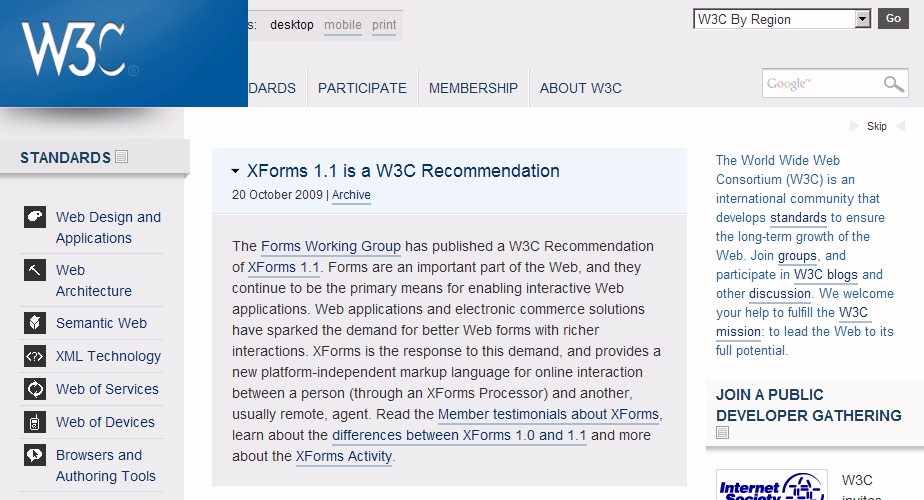This screenshot displays the front page of the W3C website, a highly recognizable resource within the web development community. In the top left corner, the website's logo, "W3C," is prominently featured within a dark blue box, slightly overlapping the menu bar. The visible portion of the menu bar includes the options "Participate," "Membership," and "About W3C," positioned to the right of the logo.

In the upper right corner, the site provides a drop-down menu labeled "W3C by region" accompanied by a "Go" button, ensuring users can easily select their specific regional site. Next to this is a search bar for efficient navigation of the site.

The sidebar begins with the heading "Standards," under which there are several items listed in sequence: "Web Design and Applications," "Web Architecture," "Semantic Web," "XML Technology," "Web of Services," "Web of Devices," and "Browsers and Authoring Tools."

The main content area features an article titled "XForms 1.1 is a W3C Recommendation,” dated October 20, 2009, and already marked as archived. The article, about a paragraph in length, is contained within a gray box.

To the right of this article, in blue text, there is a brief explanation of what the W3C is, highlighting that it stands for the World Wide Web Consortium and outlining its mission and objectives. Below this description, a small banner invites users to "join a public developer gathering.” This screenshot effectively encapsulates the structured and resourceful layout characteristic of the W3C website.